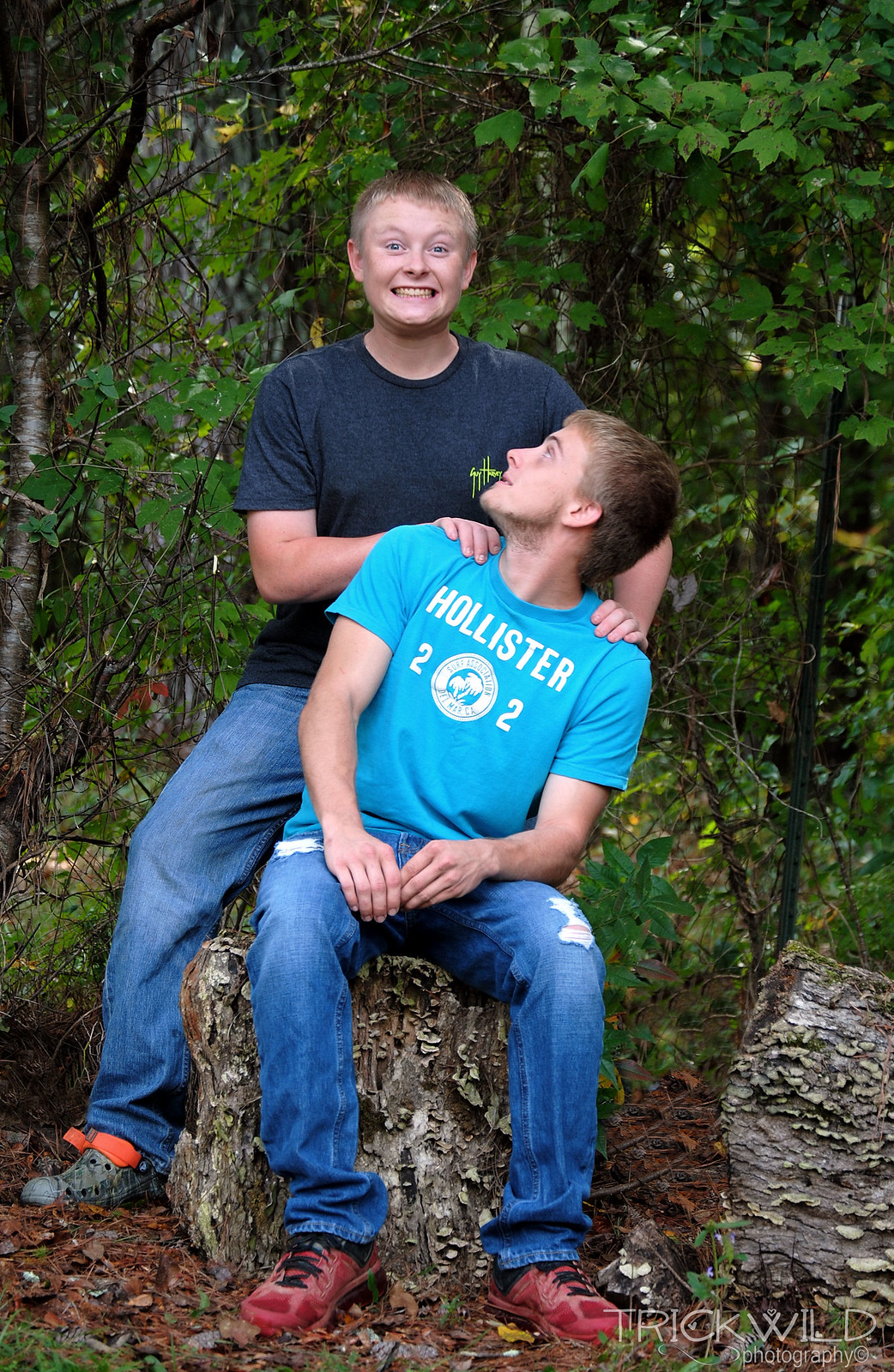In a vibrant, green wooded area, two teenage boys are captured in a moment of playful camaraderie around a tree stump. The boy seated on the stump is wearing a light blue 'Hollister 22' t-shirt, blue jeans with stylishly spaced holes, and reddish tennis shoes with black shoelaces. He has brown hair with a hint of facial hair and is looking up over his right shoulder at the other boy standing behind him. This standing boy, possibly his older brother, is straddling the tree stump with a wide, bright-eyed grin, his teeth clenched in delight. He has short blonde hair and is dressed in a dark blue t-shirt, blue jeans, and green shoes with distinctive orange straps. His hands rest on the shoulders of the seated boy as they share this joyful outdoor moment. Surrounding them is lush grass and dense trees, emphasizing the natural, wooded setting. At the bottom right of the photo, the words "Trick Wild Photography" are prominently displayed.